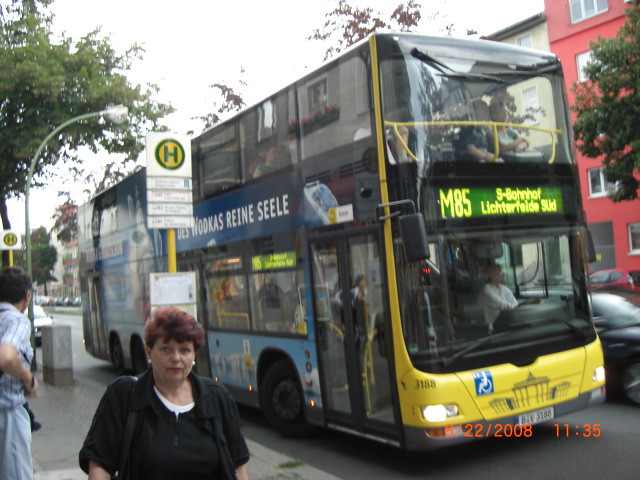This detailed photograph captures a bustling city street scene, taken on August 22, 2008, at 11:35 AM, as indicated by the timestamp in the bottom right corner. The centerpiece is a yellow double-decker bus displaying the route number M85 with a destination marquee reading "S-BAHNHOF LICHTERFELDE," written in German, suggesting the location is in Germany. The bus features large glass windshields through which the driver and several passengers are visible. The exterior is adorned with various advertisements, including one for vodka. 

In the foreground, a woman with short reddish hair, pearl earrings, and a black outfit consisting of a shirt and jacket looks directly at the camera. She carries a black bag and wears lipstick, giving her a composed appearance. To her left, a man in a blue and white checkered shirt, with glasses and a backpack, walks in the opposite direction. There's another indistinct male figure partially visible next to a tree in the background. 

Moreover, a distinct yellow signpost with an H inside a green circle further suggests this is a bus stop. The backdrop includes a salmon-colored brick building, likely residential. The combination of these elements provides a rich, contextual snapshot of daily urban life, likely in Germany.